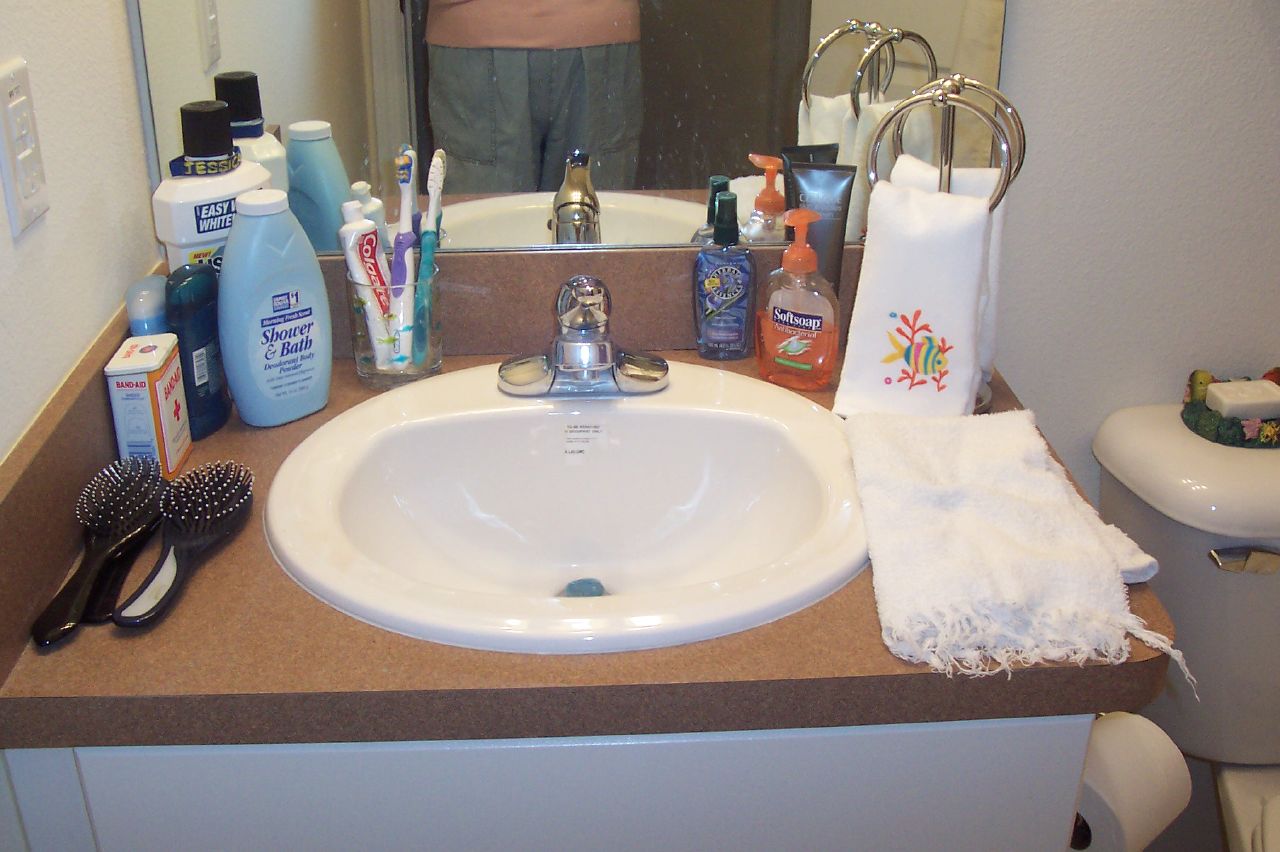In this home bathroom scene, the focus is on a spotless white sink with sleek silver hardware, set against a tan brown countertop. The counter is cluttered with a multitude of everyday items: two hair combs, a box of band-aids, a bottle of mouthwash, two deodorants, and a cup holding two toothbrushes and a tube of toothpaste. Also present are containers of hand soap and powder, along with a decorative towel on a small towel holder and another towel draped to the side. In the background, a mirror reflects a man dressed in grey shorts and a light peach-colored top. To the right, a toilet paper roll hangs from the side of the counter next to a partially visible toilet bowl, offering a glimpse into the functional aspects of this well-used space.